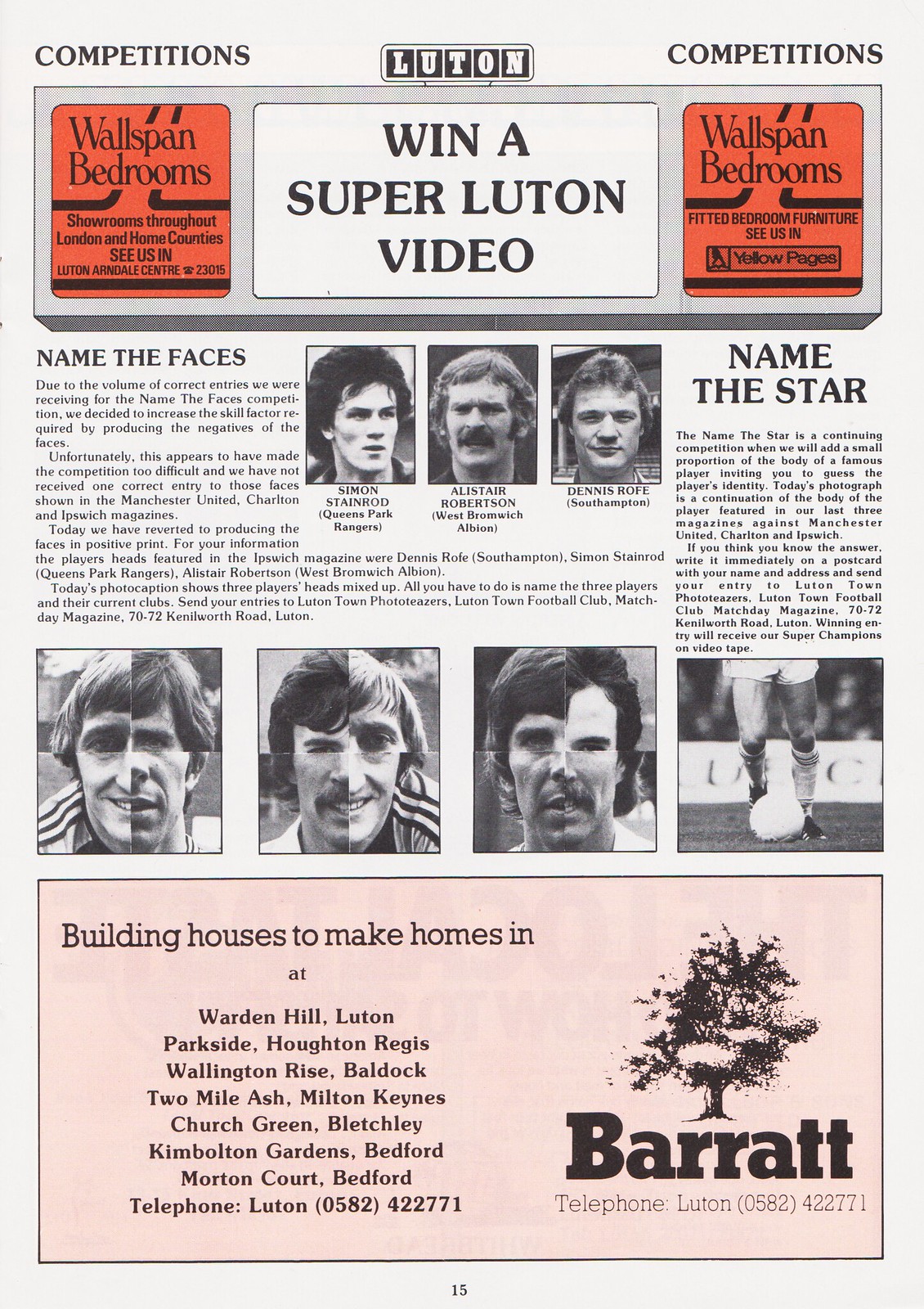This photograph captures an advertisement from a magazine with a complex and detailed layout centered around a football-themed competition. The image features a beige background and bold black text reading “Competitions” across the top. The headline “Win a Super Luton Video” stands out prominently within a white rectangular box framed by orange panels with the words "Wall Span Bedrooms" in black text. This central panel sits on a gray background, and both orange panels mirror each other.

The heart of the image focuses on a competition where participants are challenged to name the heads of football players from various clubs. The ad explains that due to too many correct entries in previous competitions, the magazine had opted to use negative images of faces, but this resulted in no correct submissions. Consequently, they reverted to using positive prints of the three players. A detailed notation mentions that the heads featured in the Ipswich magazine were Dennis Roof from Southampton, Simon Stainrod from Queen's Park Rangers, and Alistair Robertson from West Bromwich Albion.

Below the main competition text, there is a grid-like layout showing images of three football players’ faces in the middle section, requiring participants to identify them and their current clubs and send their entries to Luton Photo Teasers, Luton Town Football Club, Match Day magazine.

At the bottom, a light pink segment spans across the page, featuring an advertisement with the slogan “Building Houses to Make Homes,” listing several town names, and branding from Barrett, alongside a stylized tree image in black ink. The page number, either 13 or 15, is visible at the bottom.

Overall, this multi-layered ad combines a sports-themed challenge with a detailed layout of text and images, clearly designed to engage football enthusiasts in a skill-based competition.